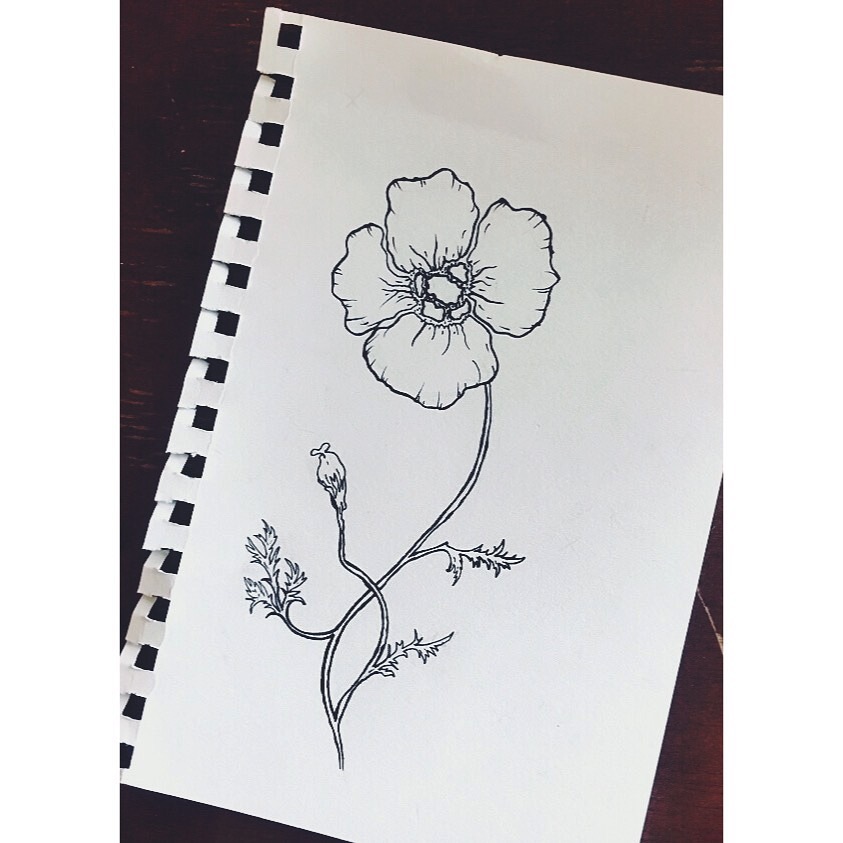This is a detailed sketch of a single blooming flower on a white, unlined piece of notebook paper, with a perforated edge visible on the left where it was torn from the notebook. The illustration, created with a fine black pen, looks almost like a printed image. The central flower has four large and irregularly shaped petals with a ring of dark spots in its imperfectly circular center. Extending from the winding stem are three shorter stems, each bearing a leaf, and one features an unopened bud. The paper is set against a dark brown wooden table, with the wood grain running horizontally across the background.